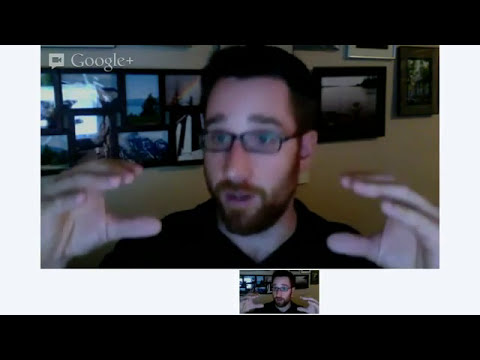The image shows a man with short, brown hair, a well-groomed beard, and a goatee, wearing black-rimmed glasses and a black shirt. He appears to be on a Google Plus video call, as indicated by the Google Plus logo in the upper left corner. The room he's in has white walls adorned with black-framed pictures, showcasing various ocean and mountain sceneries. The main picture of the man dominates the upper part of the screen, with a smaller, white-bordered version of the same image below. The man’s facial expression is slightly stunned, with his mouth slightly open and his eyebrows raised. His hands are positioned in front of him, forming a cupped shape. The room is dimly lit, giving a dark background contrast to the white walls. One of his ears is visible, and behind him, the image frames have details like smoke rising and lake views.